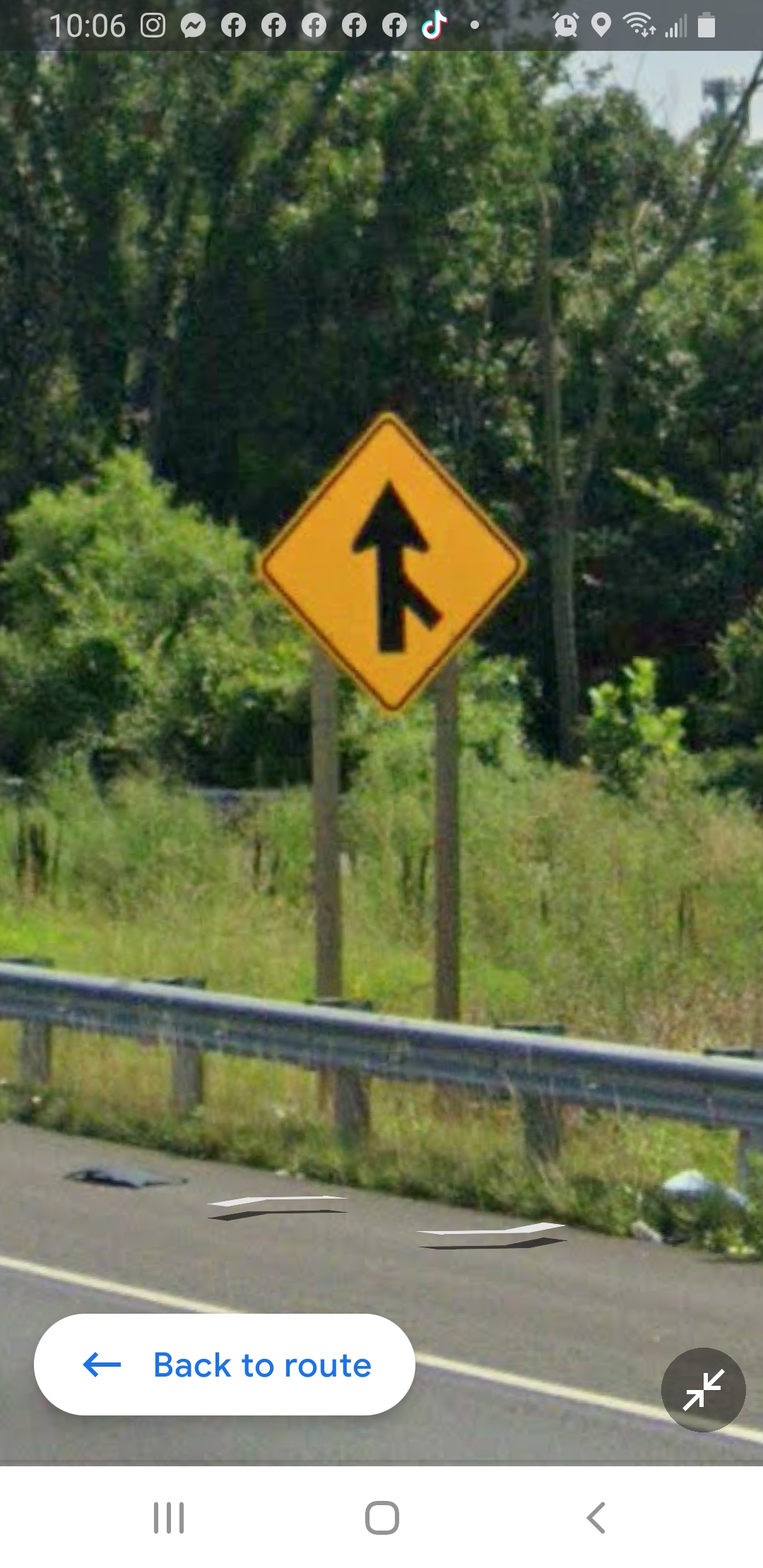This detailed caption is a refined description of the image captured:

"A screenshot of a smartphone display showcases the Google Maps app, or a similar navigation tool, with the screen zoomed into the Street View of a route. In the upper right corner, the time reads 10:06. Surrounding the time are several app icons, including numerous Facebook icons, as well as TikTok and Instagram. The upper right side displays a strong Wi-Fi signal, an active alarm bell icon, and a nearly full battery indicator.

Dominating the screenshot is a Street View image of a highway. The primary focus is a yellow diamond-shaped traffic sign featuring a black arrow pointing upwards with a smaller branch extending from the bottom right of the arrow, warning of a merging road ahead."